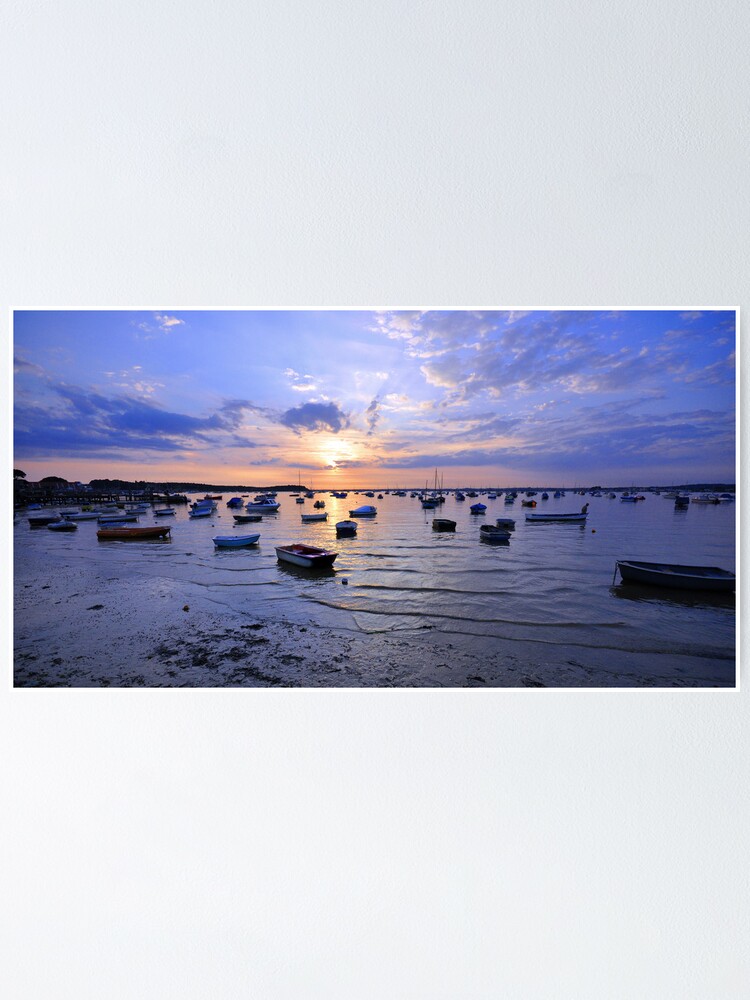The image captures a serene coastal scene at either sunrise or sunset, bathed in hues of deep blue, yellow, and orange. The expansive sky, adorned with both fluffy and darker clouds, transitions seamlessly into a warm yellowish-red near the horizon, where the sun sits low, casting its glow. In the foreground, a sandy beach meets the gentle laps of the ocean's edge. Scattered across the tranquil water are numerous small and medium boats, including rowboats, positioned in various directions and appearing empty. The scene is further enriched by the presence of subtle mountainous mounds on the left side of the horizon, enhancing the overall natural beauty. The combination of vivid colors and precise details suggests a composition that could be the work of a professional photographer.